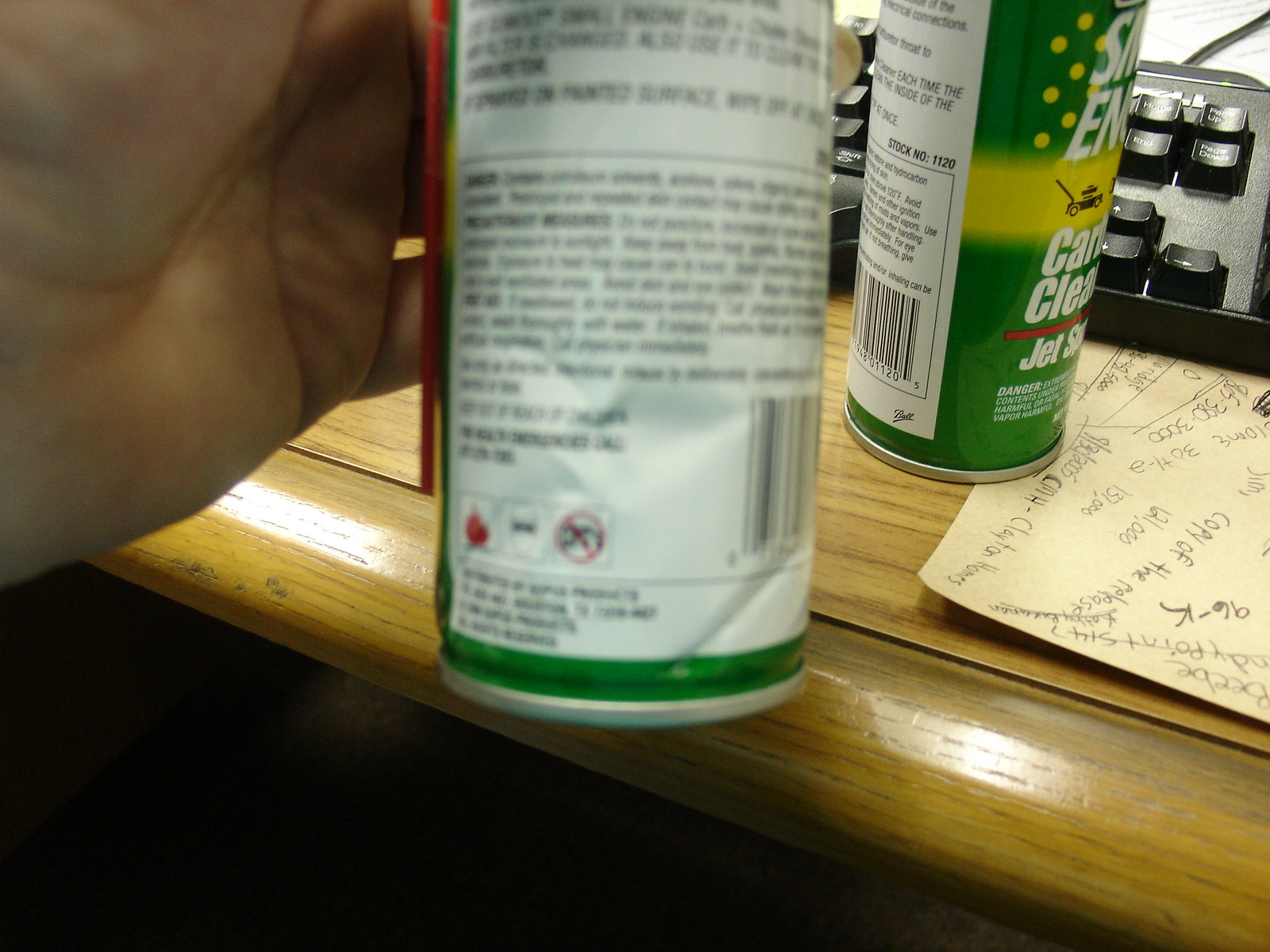The image depicts a person's left hand, palm facing the camera, holding a canister above a wooden desk. The canister label is blurry but appears to have letters "S-M" and "E-N," possibly indicating a product with "enamel" in the name. The hand appears positioned to display the back of the can, where safety instructions or ingredients are printed. Notably, this canister is equipped with a red plastic tube taped to its side, suggesting it's a spray can, potentially used for detailed applications like cleaning or painting. 

In the background, another similar can rests on the desk, featuring a notable yellow stripe around its label. The label on this can, although indistinct, bears the words: "C-A-R-T," "clean," "jet," and another word starting with an "S," hinting that the product could be a cleaner, possibly a carburetor cleaner, reinforced by the presence of a lawnmower image on its label. The background includes a black keyboard situated on the desk, partially covering a piece of paper filled with writing and numbers, underlining a context of workspace or maintenance activity. This combination of elements suggests the person might be using the can to clean their keyboard or other equipment.